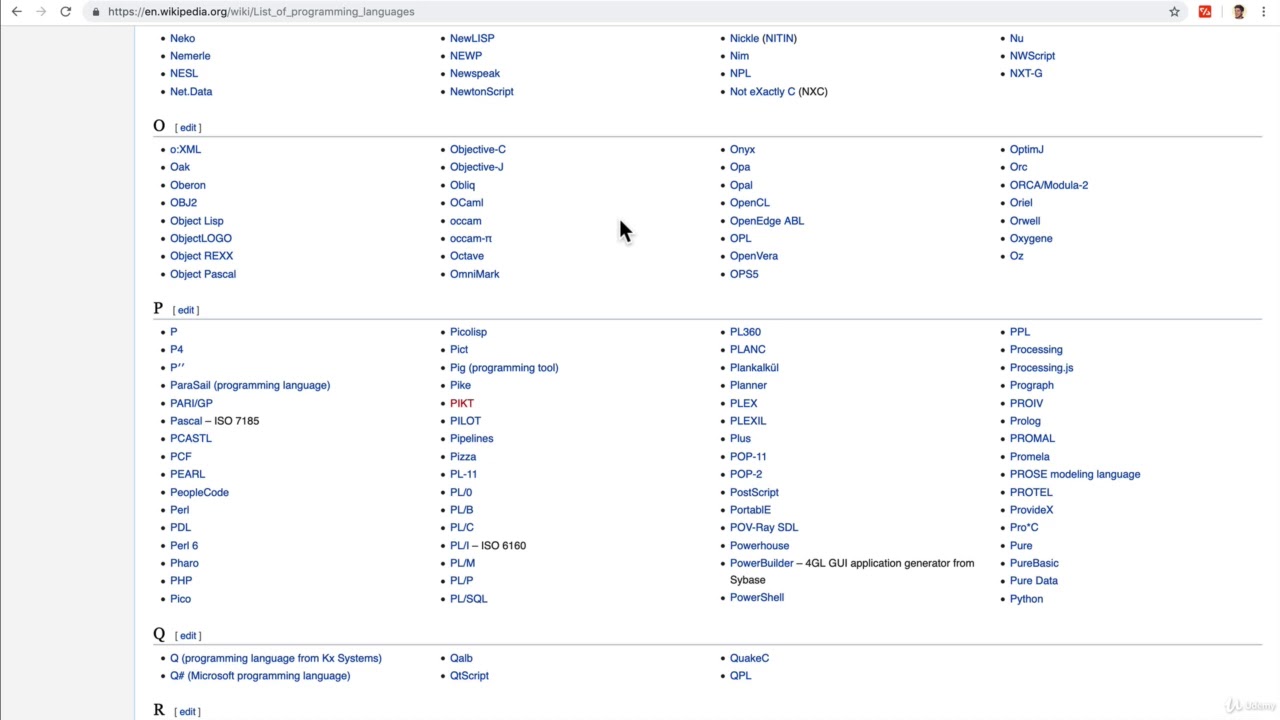The image depicts a Wikipedia page listing various programming languages. The view is focused on languages starting from the letter N to the letter R. Specifically, it partially shows some languages beginning with 'N', includes all languages starting with 'O', all of 'P', all of 'Q', and only one of 'R'. 

The languages are displayed in a vertical list, each preceded by a black dot, with each language name rendered in blue, indicating that they are clickable hyperlinks leading to their respective Wikipedia pages. Examples under the letter 'O' include O.XML, Oak, Oberon, OBJ2, and ObjectLISP. The alphabetical section 'P' features a notably extensive list of programming languages compared to the others.

This organized and hyperlink-rich list serves as a comprehensive catalog of programming languages, accessible through the alphabetic letters from N to R as displayed in the image.